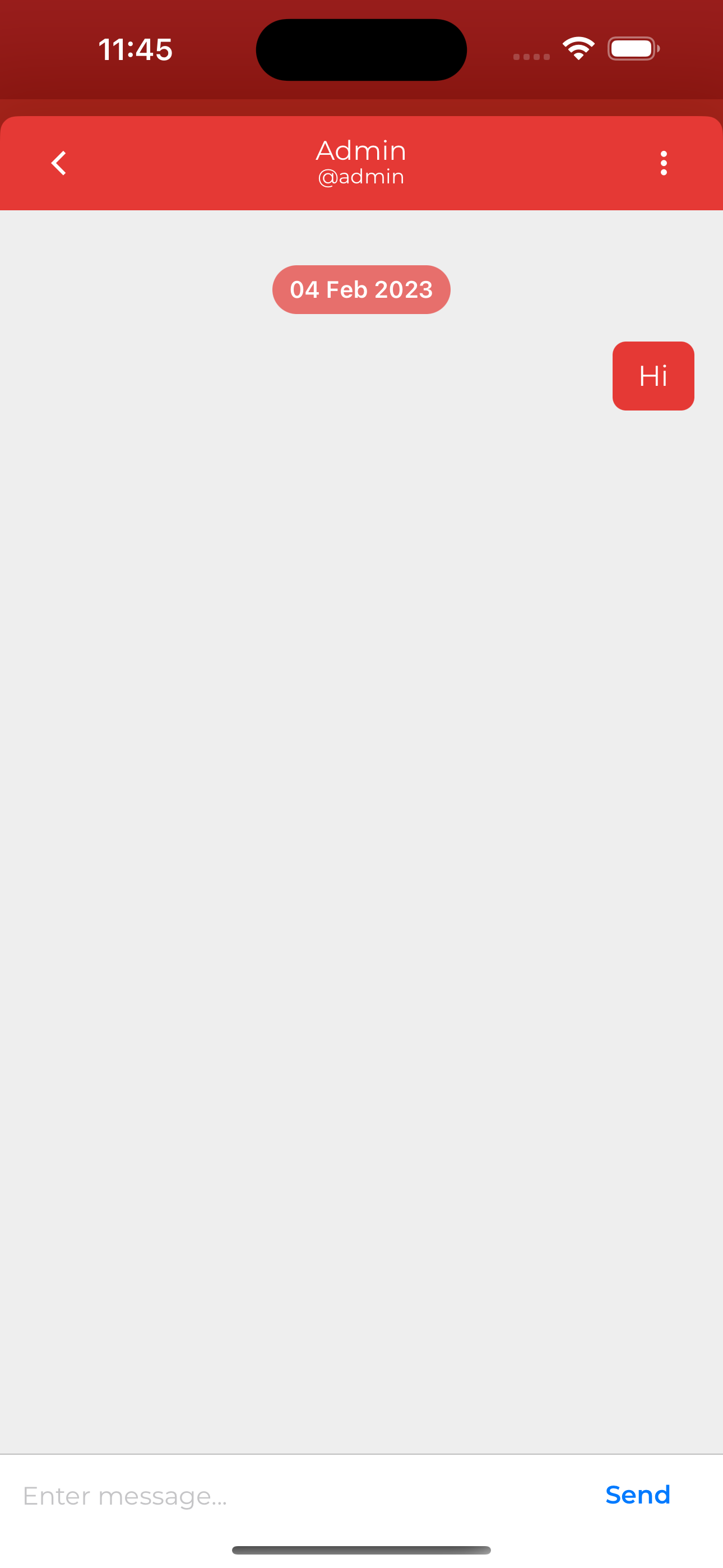A screenshot of a mobile website interface features a maroon top header with a black bubble redacting the central text. The left side of the header displays the time "11:45," and the right side shows icons for cellular signal and a full battery. Directly beneath the header is a crimson red tab containing the text "admin at admin" centered, a left-pointing arrow on the left side, and three vertical dots on the right side. Below this tab is a blank page. Near the top of this blank section is a red bubble labeled "February 2023." Further down on the right side is another red bubble with the word "Hi" in white text. At the bottom of the message box, there is an input section labeled "Enter message," and to the right of this section is a blue "Send" button.